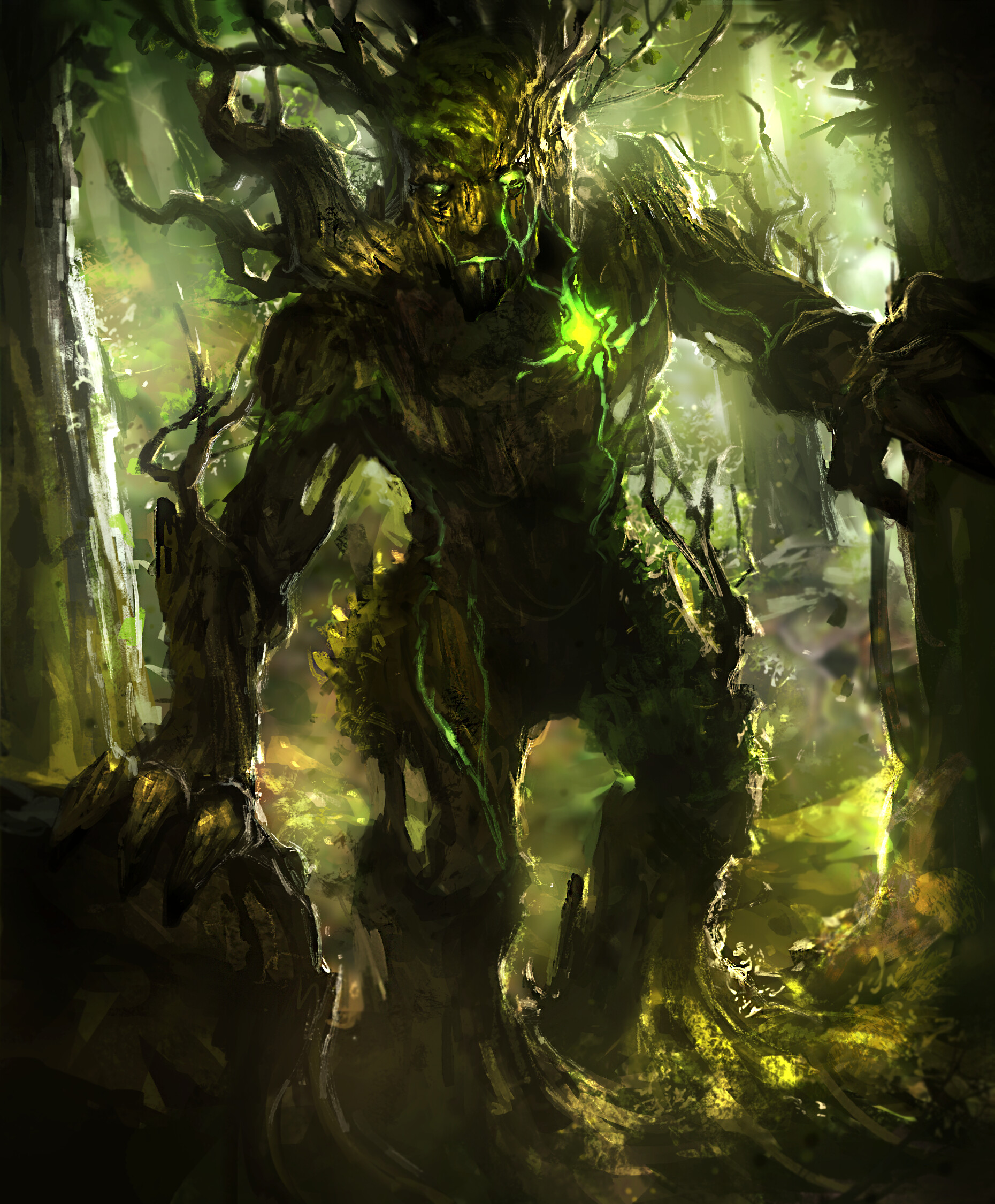This image, reminiscent of a horror movie or video game, features a terrifying, tree-like creature standing ominously in a forest. The creature's body appears entirely composed of dark tree trunks and branches, with neon green highlights casting an eerie glow. Its menacing face, complete with small, glowing green eyes and a similarly luminescent mouth, is carved from what looks like twisted branches. Branches even protrude from its head and back, emphasizing its monstrous, arboreal nature.

The creature's limbs resemble the trunks and limbs of trees, its feet rooted like actual tree trunks with smaller branches jutting out. One of its claw-like hands is placed firmly on a large, dark rock in the foreground, while the other touches a nearby tree, enhancing its menacing presence. In the area where its heart would be, a pulsating, neon green glow emanates, adding to the monstrous allure.

The background features a dimly lit forest, with regular trees on either side of the creature. The forest is bathed in a murky green light, interspersed with patches of yellow-neon hues, contrasting sharply with the dark, shadowy areas, and creating a dappled, unsettling atmosphere. This eerie scene, paired with the creature's formidable stance, makes for a visually striking and haunting image.